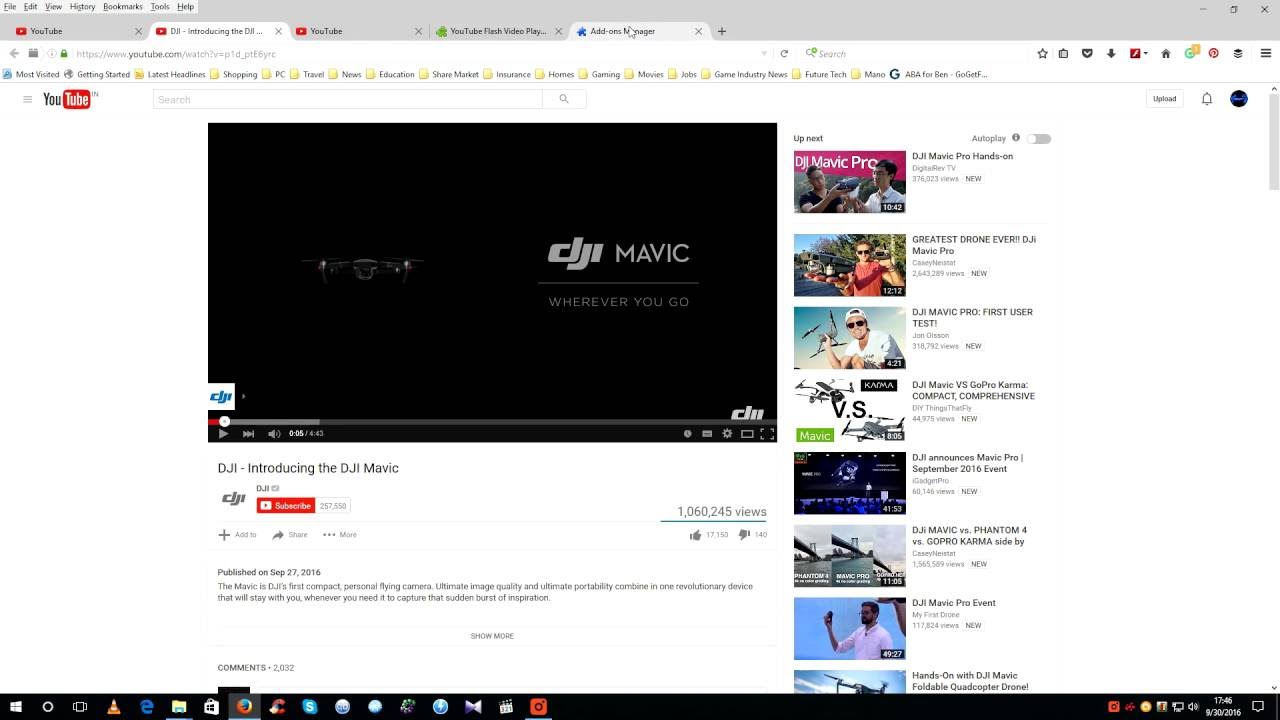A screenshot captures a YouTube video being watched on a computer. The video, titled "DJI introducing the DJI Mavic," features a tagline on the screen that reads, "DJI Mavic: wherever you go." The video appears to be highly popular, having garnered over a million views. 

The YouTube sidebar showcases a series of related videos, predominantly highlighting various aspects of the DJI Mavic drone. The suggested videos include titles such as "The Greatest Drone Ever," "DJI Mavic vs. Phantom 4," "DJI Mavic Pro Karma Contact Comprehensive," "DJI Mavic Pro Hands-On," "DJI Mavic Pro First User Test," "DJI Announces Mavic Pro," "DJI Mavic vs. Phantom 4 vs. GoPro Karma Side-by-Side," "DJI Mavic Pro Event," and "Hands-On with DJI Mavic Foldable Quadcopter Drone." Each of these suggested videos features detailed reviews, comparisons, and user experiences with the DJI Mavic drone lineup.